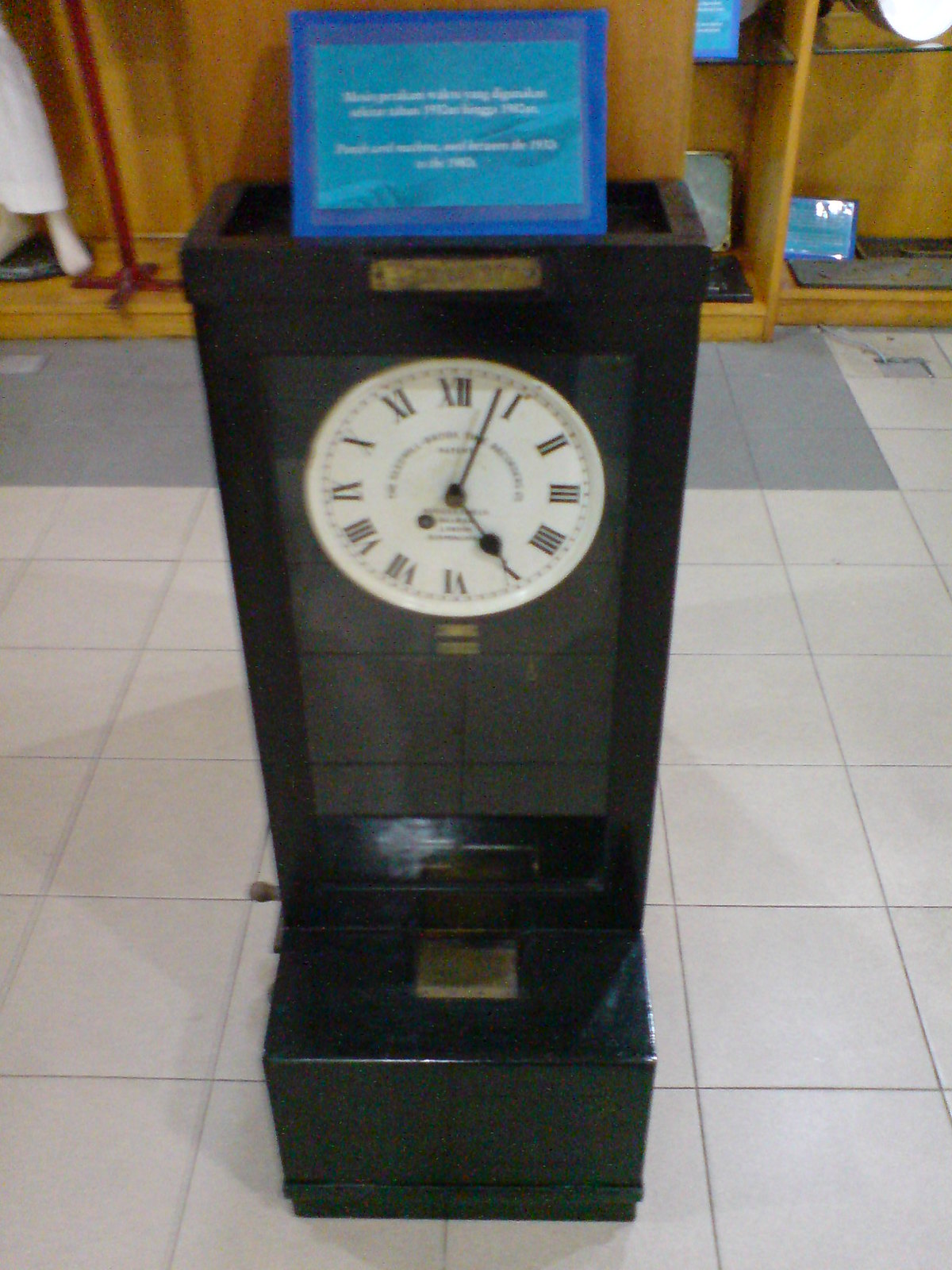The photo appears to be taken inside a museum, providing a bird's-eye view of an intricately detailed display featuring an old-fashioned grandfather clock. The clock, which is black, has a tower-like structure with a flat top. Prominently displayed on its front is a gold label. The clock boasts a glass window that reveals a white clock face adorned with Roman numerals, with the time indicating 5:03. This elegant timepiece stands on a black base that could be part of its original design, and this base features another gold square, possibly containing a carving that remains indistinct due to the photo's blurriness.